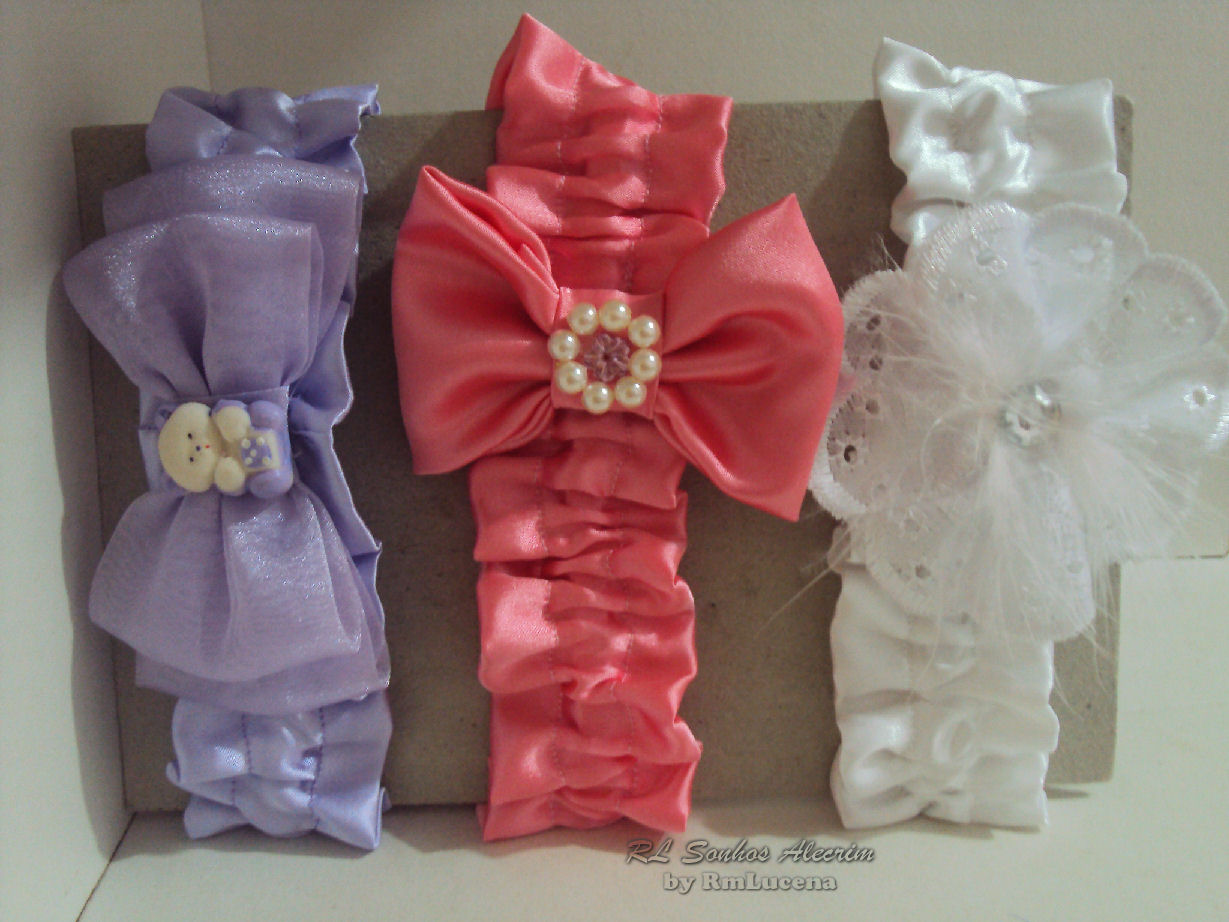The image depicts a product photograph showcasing three decorative headbands arranged on a piece of light gray cardboard. Each headband is made from a stretchy or satin material and features distinctive embellishments. The headband on the left is lavender with a fabric bow adorned by a small white bear charm at the center. The middle headband is a hot pink or salmon color, highlighted by a floral pink button encircled by white pearls. The rightmost headband is white, decorated with a lace flower that has white wisps or feathers extending from it, and a silver or clear gemstone in the middle. The headbands are neatly displayed against a light gray background. Encapsulated within a white box, the bottom of the photograph includes text reading "R.L. Solos Alcerin by R.M. Usaino," though slightly illegible. The overall style of the image is photographic realism.